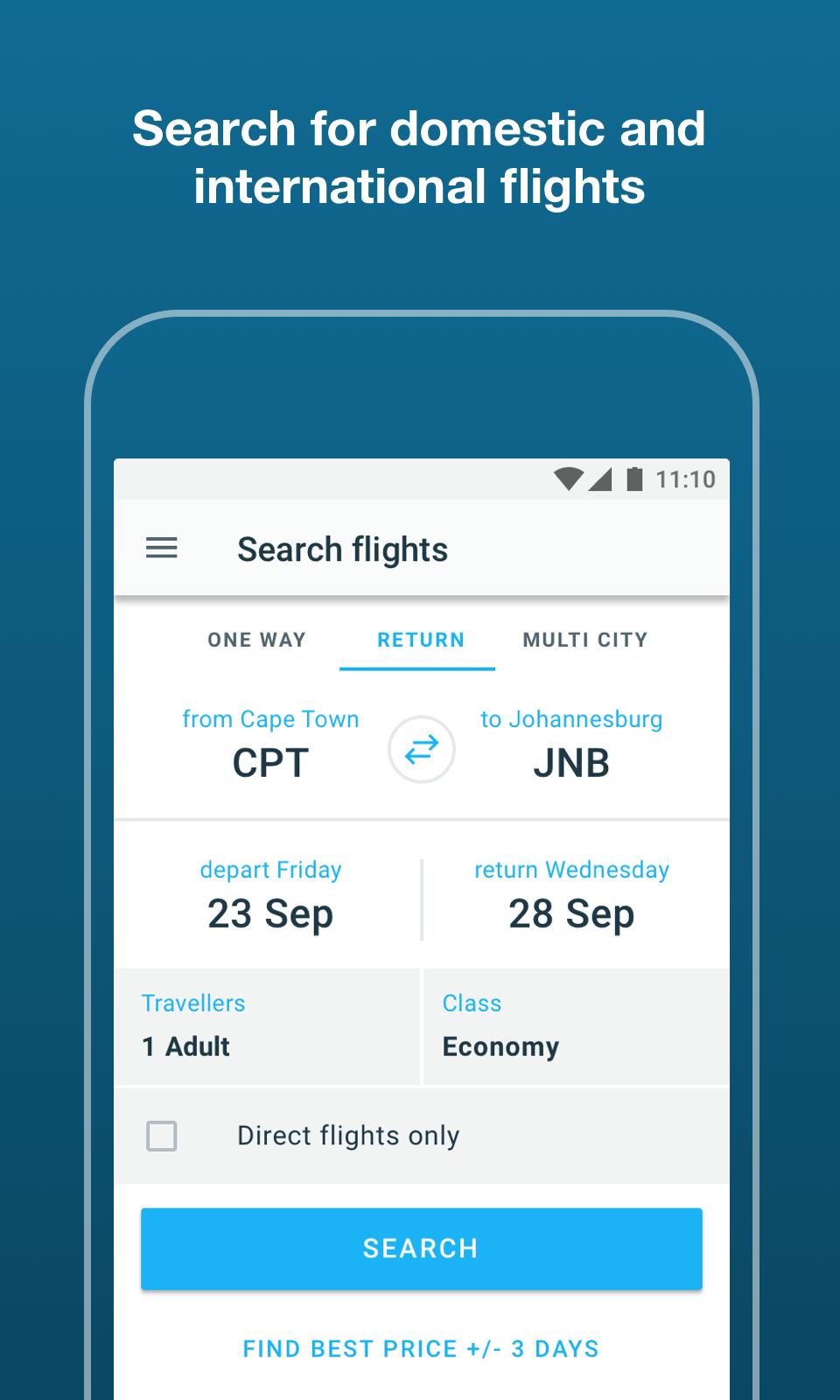The image depicts a search interface for domestic and international flights, set against a blue background. Central to the design is an illustration of a smartphone, guiding users on how to look for flights. At the top of the screen is a search box labeled "Search for flights" with options for one-way, return, or multi-city trips. In this instance, the "Return" option is selected. The chosen route is from Cape Town to Johannesburg, with the departure date set for Friday, September 23rd, and the return date for Wednesday, September 28th.

Beneath these fields, users can specify the number of travelers and the travel class; here, one adult traveler has been selected for economy class. Additionally, there is an option to filter for direct flights only, though this box remains unchecked. A prominent light blue search button is positioned below these options, ready to initiate the flight search. For more flexible travel plans, there's a feature that allows users to find the best prices within three days before or after their selected dates. Despite the lack of branding information, the clean and intuitive design effectively guides users through the flight search process.